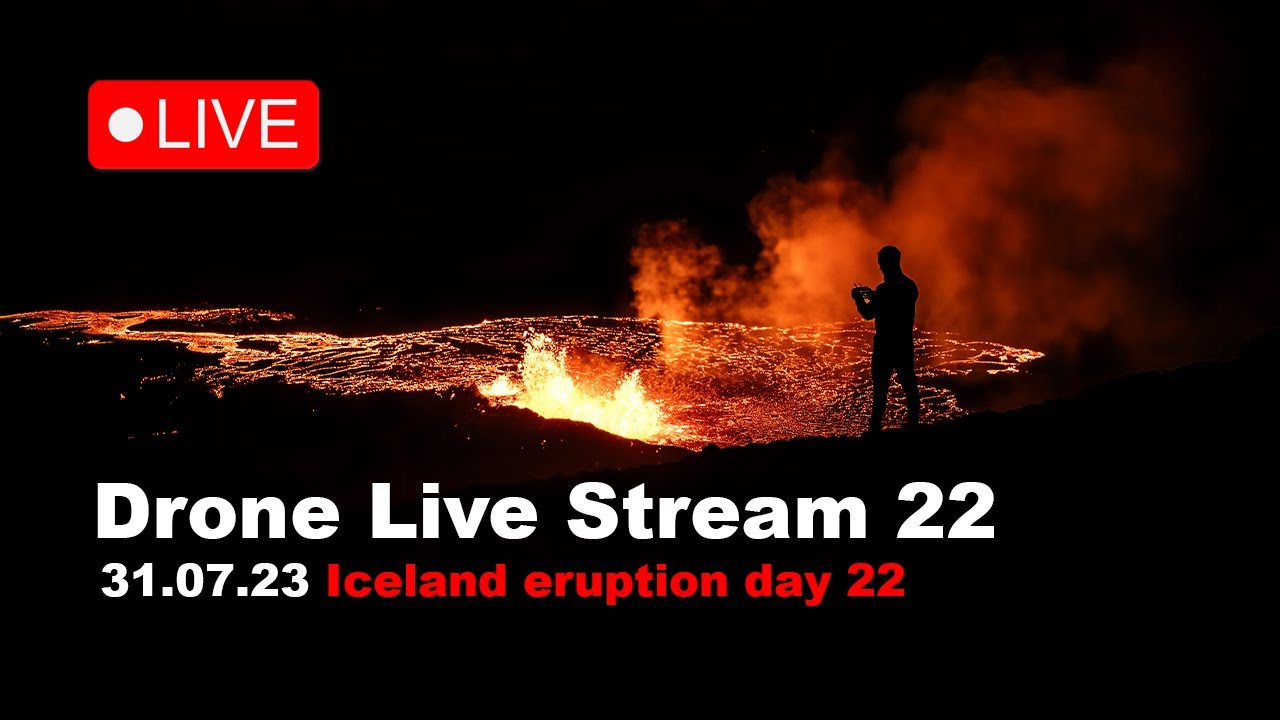At night, an outdoor photographic image captures a man standing with his back to the camera on the edge of a volcanic eruption. His silhouette contrasts dramatically against the illuminated sky. He's holding what appears to be a cell phone, looking downward at the widespread orange lava and the billowing orange smoke. The scene is set against a dark, rocky landscape, with most of the image dominated by the fiery eruption. In the top left corner, text in formats of white on red and white on black reads "Live" and "Drone Livestream 22," along with "31.07.23" and "Iceland Eruption Day 22," marking the ongoing event's 22nd day.